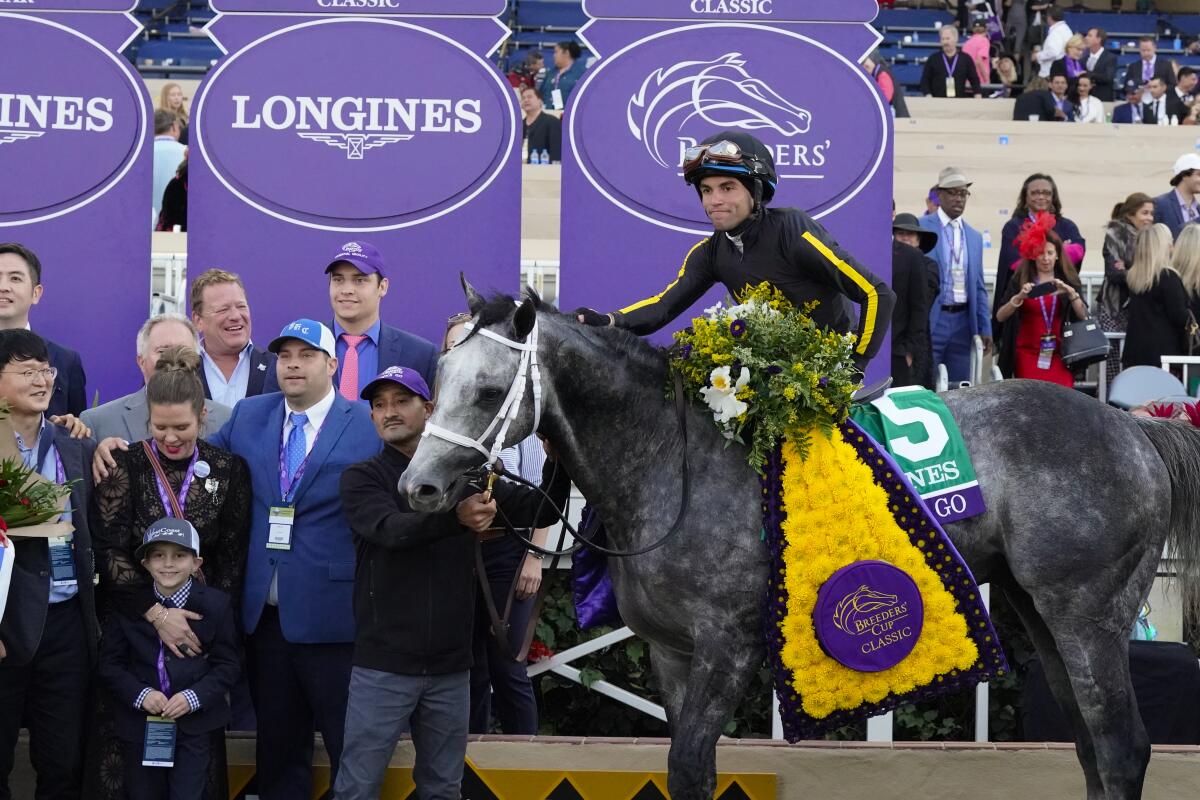In the winner's circle at the end of a horse race, this vibrant photograph captures a jubilant scene centered around a striking splotchy dark gray and light gray horse with a prominent white mark on its forehead. The horse is adorned with a white bridle and black reins. Atop the horse sits the triumphant jockey, whose black jersey sports distinctive yellow stripes down each arm. The jockey, wearing a black helmet with goggles perched on top, radiates a satisfied smile. His torso is draped with a lush garland of flowers, partially obscuring his figure.

A gentleman stands proudly beside the horse, holding the reins and posing for the celebratory photograph. In front of the jockey, emerging from the floral arrangement, is a prominent pyramid-shaped object primarily yellow with blue borders and emblazoned with the Breeders' Cup Classic seal. The background features a stanchion adorned with advertisements, prominently displaying the names "Longines" and "Breeders." Surrounding the central figures are various individuals, young and old, men and women, all smiling and sharing in the victorious moment. Red banners further frame the festive atmosphere, and beyond them, stands filled with spectators add to the sense of grandeur at this prestigious event.